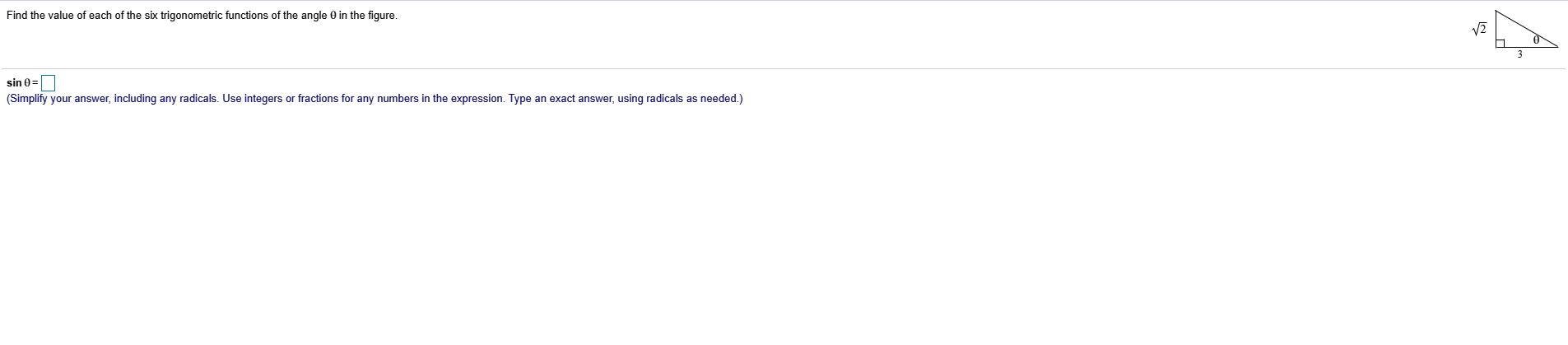This image depicts a math problem, specifically a trigonometry exercise, that might typically be encountered in a homework assignment. The problem is presented with the following instructions: "Find the value of each of the six trigonometric functions of the angle \(0^\circ\) in the figure." Below this directive, there is space provided for answers under prompts such as "sin(0) =", with an additional note in parentheses: "Simplify your answer, including any radicals. Use integers or fractions for any numbers in the expression. Type an exact answer using radicals as needed."

The layout of the page includes black text on a white background. The specific guidance within parentheses is highlighted in blue text for emphasis. The right side of the image features a geometric figure, including a triangle with various labeled values. There is also a degree measure marked in the inner right corner of the triangle and a part of a square visible in the lower left corner of the figure.

This problem falls within the scope of a trigonometry class, where students are expected to work with shapes and understand different angles and their associated trigonometric functions.